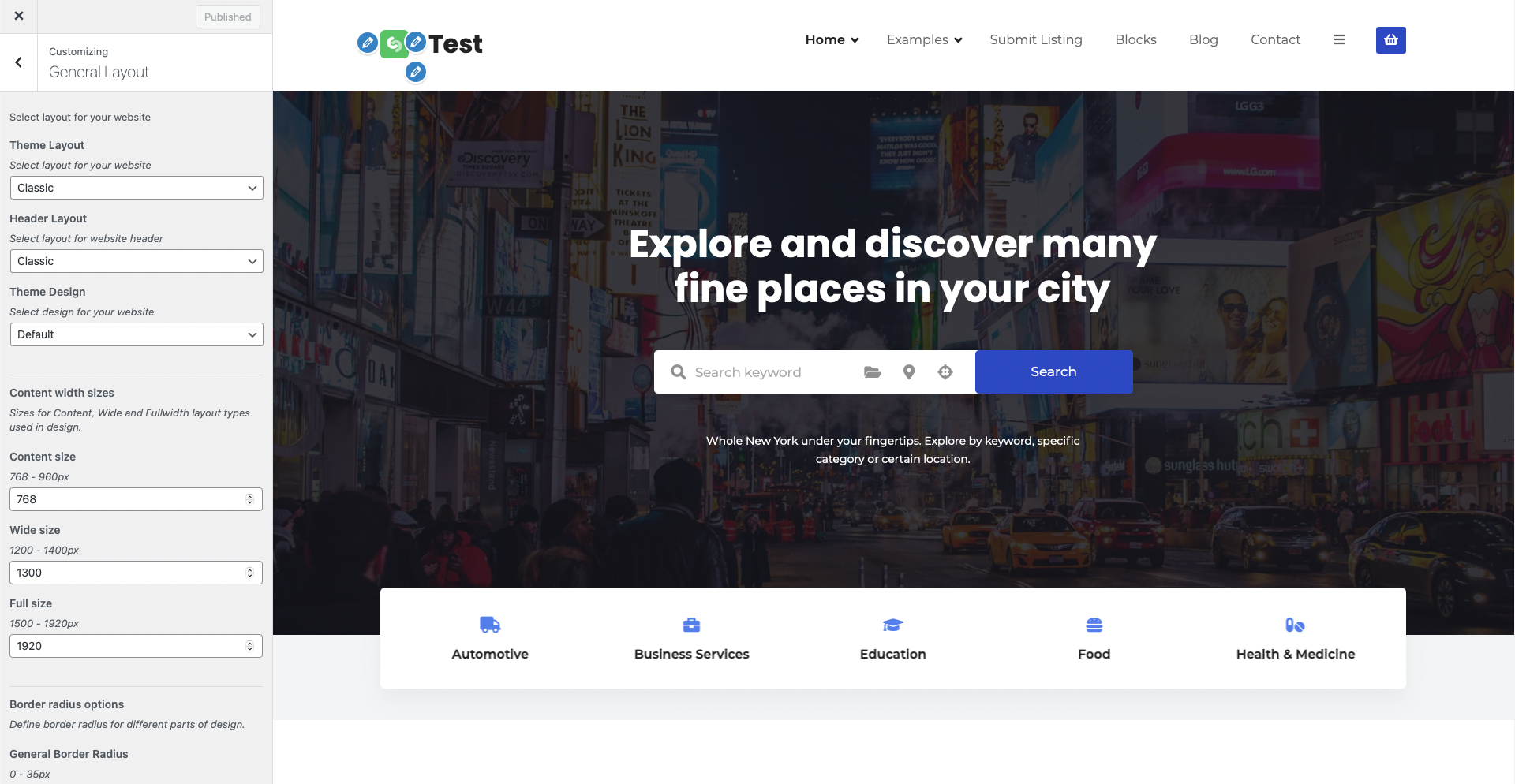This image captures a screenshot of a webpage showcasing various navigational and customization options. At the top, there is a menu bar presenting several links: "Home," "Examples," "Submit Listing," "Blogs," "Blog," "Contact," "Menu Bar," "Navigation Bar," "Customization Bar." Moving down the page, there appears to be a section dedicated to layout customization, with categories such as "Published," "Customizing," "General Layout," "Select Layout for your Website," "Theme Layout," and "Select Layout for your Website." Within these categories, there is an option labeled “Classic.” 

Following this, there is another part titled "Header Layout," with a subsequential option to "Select Layout for your Website Header," including another "Classic" style. The next segment is marked "Theme Design," proposing to "Select Design for your Website," and highlighting a design tag labeled "Divorce." 

Additionally, there is a portion addressing "Content with Sizes," providing specifics about "Sizes for Content," and the different types of layout: "Wide and Full Width Layout Types Used in Design." Detailed size options are provided: "Content Size 768," "Width Size 1300," and "Full Size 1920." This meticulous breakdown offers users a comprehensive look at the customizable elements available for their webpage design.